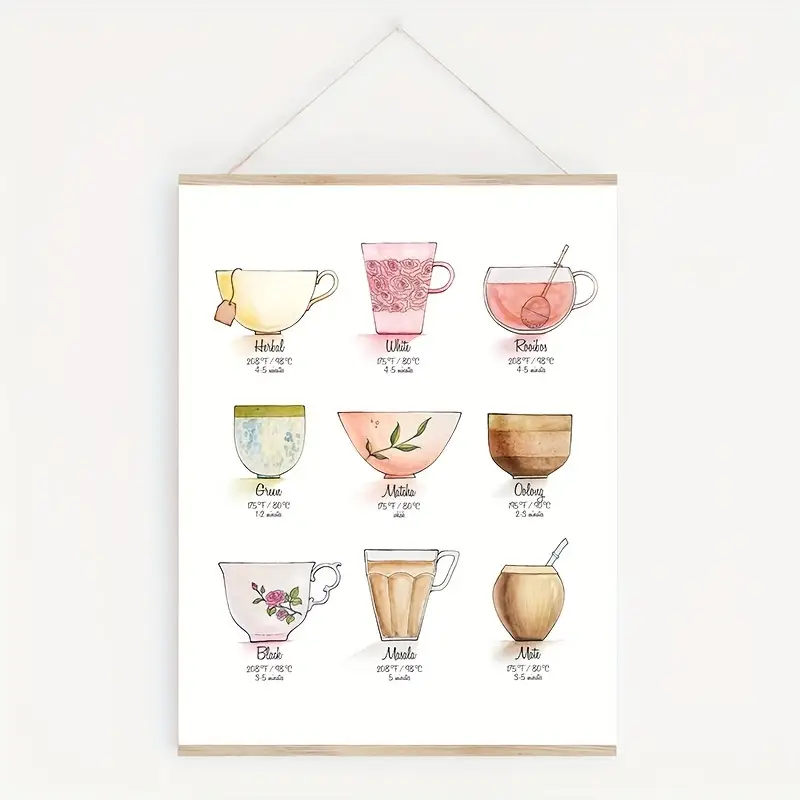The image displays a wall chart hanging from a string on a white wall, framed by two strips of wood at the top and bottom. The chart showcases nine different types of tea, each depicted in a unique cup. The teas include Herbal, White, Rooibos, Green, Matcha, Oolong, Black, Masala, and Mate. Each tea cup features specific brewing instructions, detailing the ideal water temperature in both Fahrenheit and Celsius, and the steeping time required. For example, the Herbal tea is best brewed at 208°F (98°C) for 4-5 minutes, while the Oolong tea requires 195°F (90°C) for 2-3 minutes. Some cups show tea bags, tea balls, or even a straw, adding to the variety and informational aspect of the poster. Despite some difficulty with the curvy font, it effectively serves as a comprehensive guide to enjoying these nine types of tea.